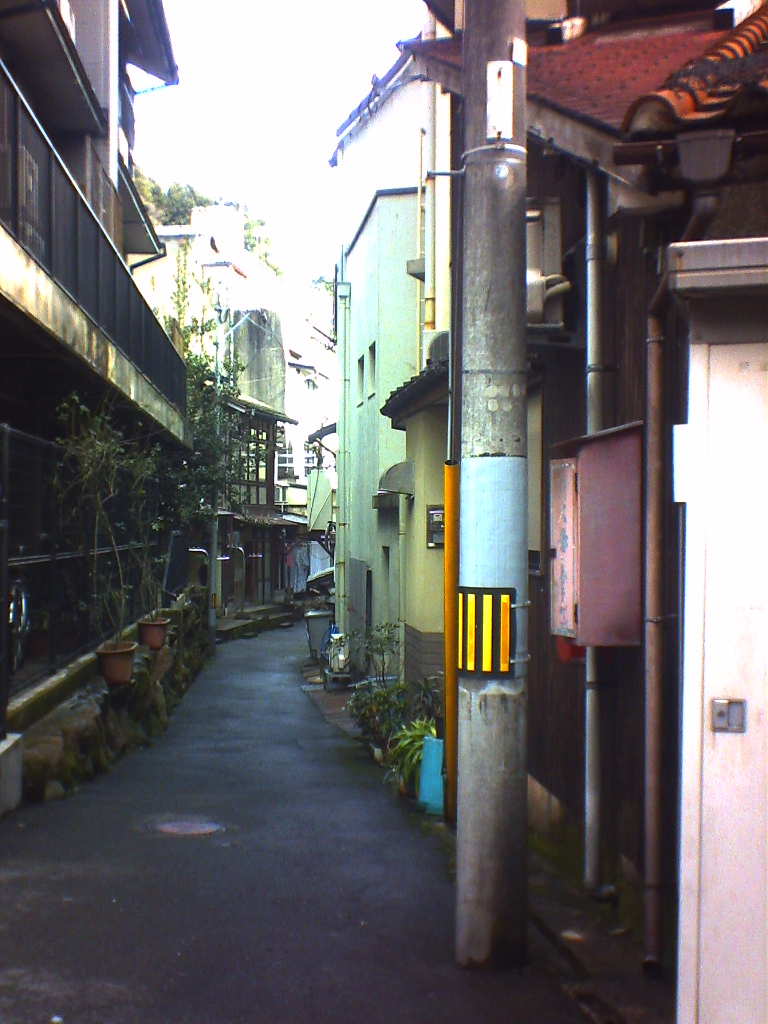This image captures a narrow, concrete walkway that cuts through a lane of diverse and colorful buildings. The path appears damp and is lined with various potted plants, bushes, and small trees on both sides. To the left, a stone fence starts at roughly 16 inches tall and progressively rises to about 4 feet as it extends into the distance. Adjacent to the fence is a multi-story building featuring a second-story deck with a black gate across the exterior. This building, along with others, showcases a mix of colors, with shades of off-white and black.

On the right side, notable details include a red tile roof, showing signs of corrosion or algae. Equally eye-catching is a blue metal pole with a sign featuring yellow and black stripes. Further along, there's a lamppost, silver and slightly rusted, contributing to the industrial feel of the alley.

Scattered across the buildings are multiple pipes descending from the roofs, with a pink box attached to a wall displaying blue text. The background sky is white, framing the alleyway in a bright, diffused light that subtly illuminates the scene. In the forefront, there is also a yellow curb and a silver bike parked near the fence, adding to the everyday urban charm of this mixed-residential area.